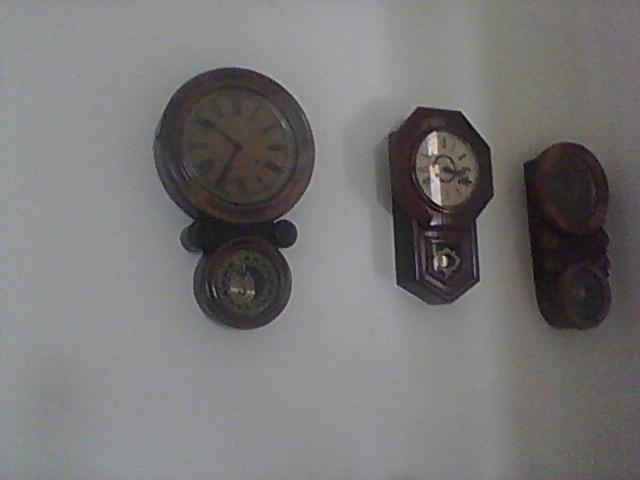The image depicts a pristine white wall adorned with three elegant pendulum clocks. Each clock features a golden pendulum encased within a wooden frame, allowing a clear view of the pendulum through a glass window. The wooden frames exhibit a rich, dark cherry wood finish.

1. The clock on the far left has a distinctive design with both a circular top and bottom. The clock face, adorned with Roman numerals I through XII, is difficult to discern but appears to be a brownish color.
   
2. The clock positioned in the middle stands out with a unique geometric form—its top is shaped like a hexagon, while the bottom takes on a triangular shape. This clock boasts a white face, also marked with Roman numerals from I to XII. There is a slight glare on its glass surface, adding a touch of brightness to the scene.

3. Finally, the clock on the far right mirrors the shape of the leftmost one, with circular elements on both the top and bottom. Unfortunately, the face of this clock is not visible.

The golden pendulums of all three clocks add a layer of sophistication and timeless elegance to the overall aesthetic.